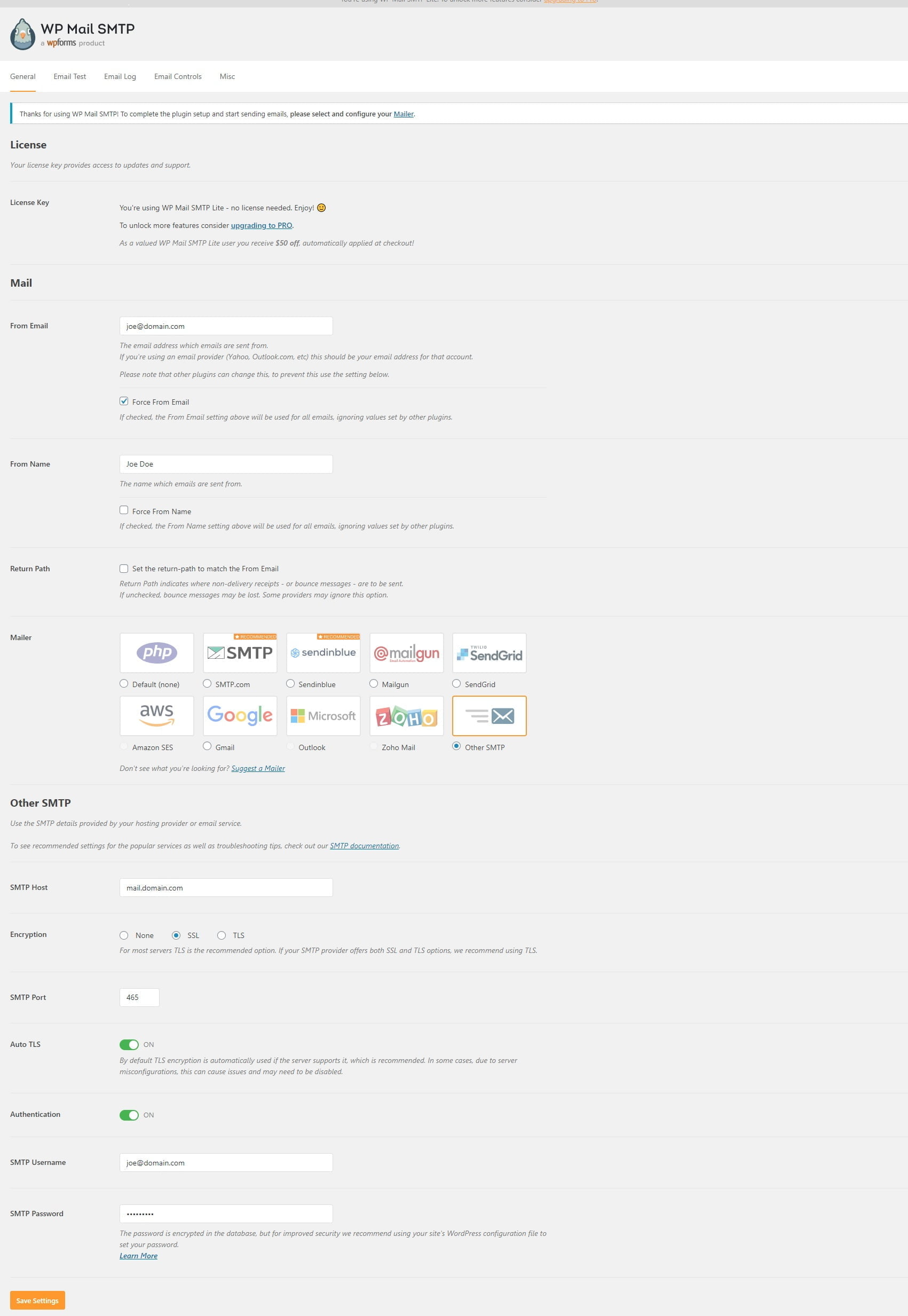In the provided image, we see the WP Mail SMTP plugin interface, a product by WP Foreigners, which features a design resembling a pigeon fade. The interface includes several menu options such as General, Email Test, Email Log, and Email Controls. 

At the top, there's an important notice advising users to select and configure their mailer to complete the plugin setup and start sending emails through WP Mail SMTP. It also mentions the licensing details, highlighting that a license key provides access to updates and support. For users of WP Mail SMTP Lite, no license is needed and they can enjoy the plugin with basic features. However, upgrading to the Pro version unlocks more features, and WP Mail SMTP Lite users can save $50 off, automatically applied at checkout.

An example email configuration shows the sender's email as joe@domain.com, which is the address from which all emails would be sent. The note suggests that if using an email provider, this should be the corresponding email address. It also points out that other plugins might override this setting but provides an option to enforce the 'From Email' setting for all emails, preventing other plugins from making changes. 

Additional options include setting the 'From Name' to ensure it is used uniformly across all emails, and specifying a 'Return Path', which indicates where undelivered receipt notifications or mail error messages should be sent.

The plugin supports various mailers, such as PHP, SMTP, Sendinblue, Mailgun, SendGrid, AWS, Google, Microsoft, Zoho Mail, and other SMTP services, providing users with a range of options to suit their emailing needs.